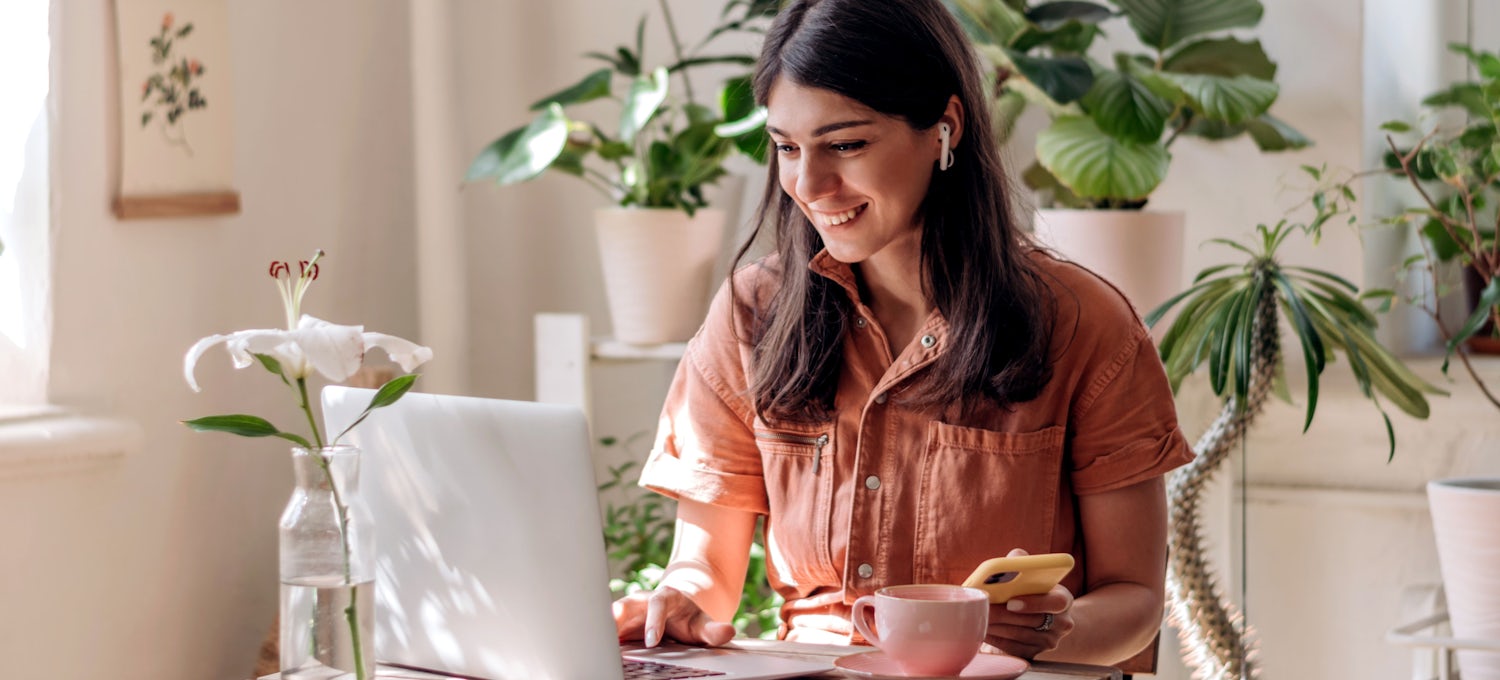The photograph, taken indoors, showcases a woman with long black hair seated at a table, engaging with her white laptop, which features a black keyboard. She is dressed in a peach-colored button-up blouse, sporting white ear pods, and brightly smiling as she types. In her left hand, she holds a cell phone encased in yellow rubber. In front of her, to the right of the laptop, rests a pink coffee cup on a small matching saucer. Behind the laptop sits a clear vase, about half full of water, containing a single white lily. The background features a white wall adorned with a picture and an assortment of green leafy potted plants, including one particularly long, curly plant trailing off-screen. To the far left, a window sill is visible. The scene is infused with a calm and productive atmosphere.